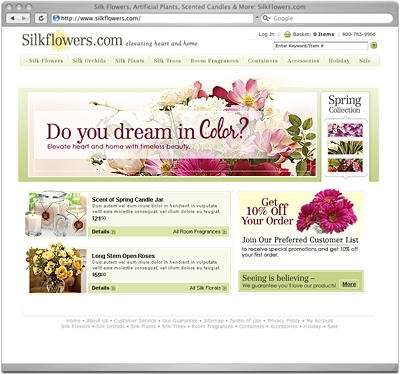This image is a screenshot of an internet browser, likely Safari by Apple, displaying the homepage of www.silkflowers.com. The webpage features a clean design with a white background, black text, and occasional splashes of red, green, and light green highlights framing certain sections. 

At the top center of the page, the website address "www.silkflowers.com" is displayed prominently in black text against the white background, accompanied by a semi-opaque yellow flower behind the word "flowers." Just beside this logo, the tagline "Elevating Heart and Home" is visible. The top navigation bar shows options to log into an account, although no specific account is logged in. There is also a shopping cart icon and a telephone number displayed.

Directly below this bar is a search function, enabling users to find specific items. The header section includes several subcategories such as "Silk Flowers," "Silk Orchids," and others that are too small to read in detail. 

Dominating the center of the page is a large, eye-catching graphic featuring a bouquet of flowers in various pinks, whites, and reds. Overlaying this image is dark crimson text reading, "Do You Dream in Color?" with the word "Color" presented in a cursive font. To the right-hand margin, there is additional text saying, "Elevate Heart and Home with Timeless Beauty," promoting their spring collection and offering different flower options.

Beneath this central graphic, several sections provide options for ordering various flowers, candles, and other merchandise. There is also a promotional text stating, "Get 10% Off Your Order," next to an image of flowers. Below this, calls to action like "Join Our Preferred Customer List" and "Seeing is Believing" are prominently displayed. The very bottom of the page contains some small, indiscernible text.